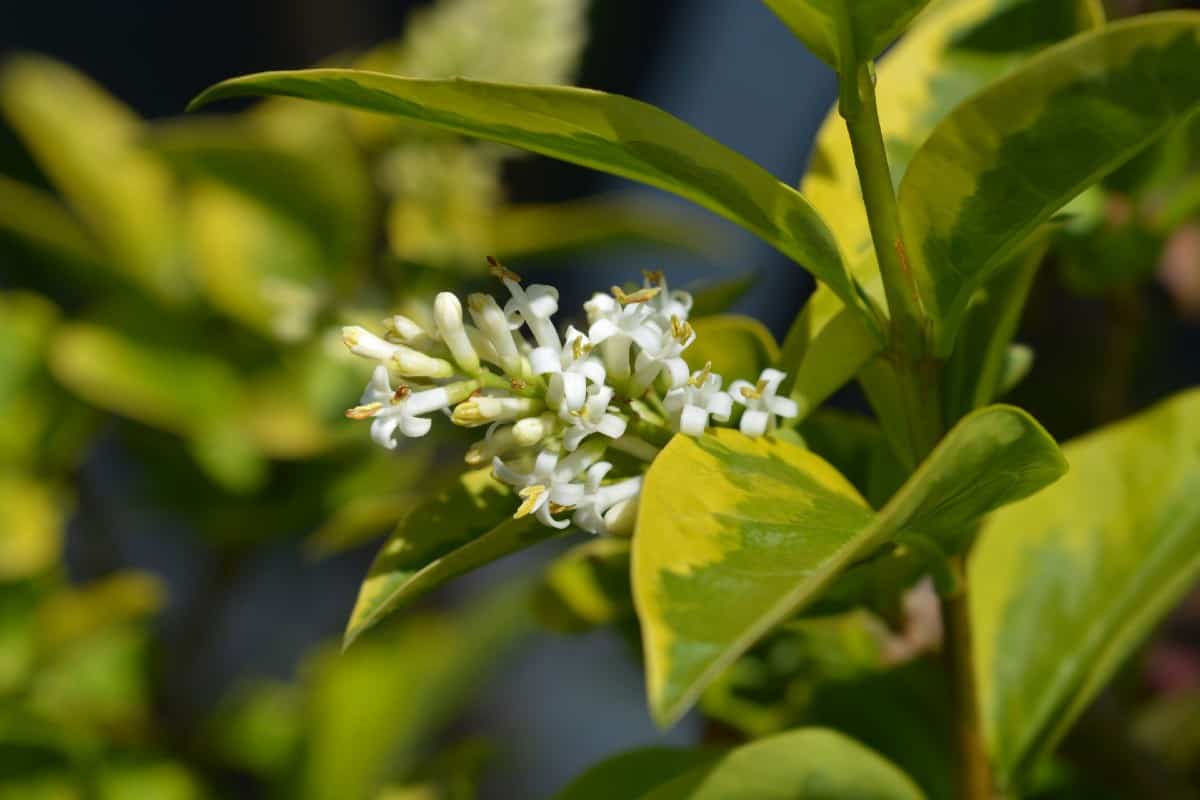The close-up color photograph captures a detailed section of a flowering plant, showcasing its various green leaves and white flowers. The leaves, which curve upward, exhibit a smooth texture and resemble triangles. They display a gradient from dark green in the center to lighter green or yellow along the edges. The plant's green stems support the leaves and a prominent cluster of white flowers positioned just behind the frontmost leaf, closest to the camera. Each small flower in this grouping appears to have four white petals with golden-yellow centers. The background is a deep, dark blue, providing a striking contrast to the vibrant greens and whites of the plant.